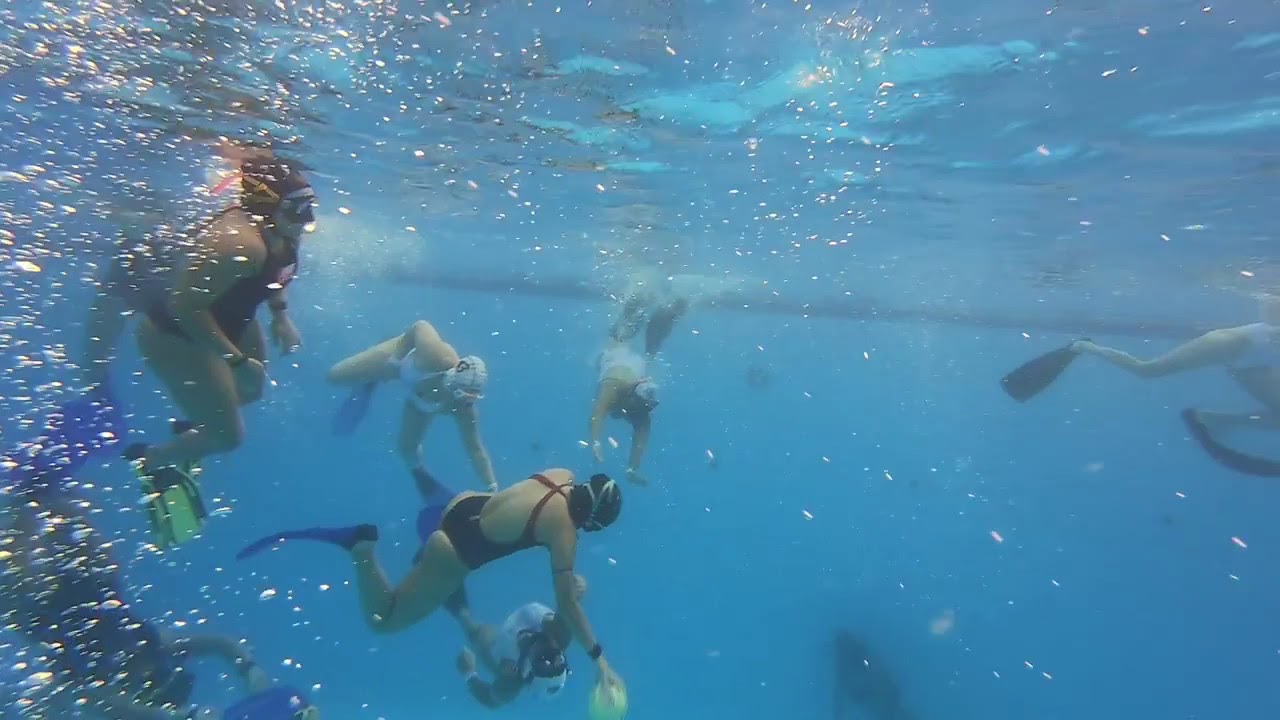The image captures an underwater scene of a water polo game held in a swimming pool. The water is a vibrant blue, with bubbles dispersed throughout, indicating movement and breathing from the swimmers. Seven female players are visible, all adorned in one-piece swimsuits in various colors—white, red, and black—and equipped with swim caps and goggles. The photo prominently features the bottom of the pool's surface and the distant, blue-tinted pool wall. In the forefront, teams are distinguishable by their differently colored gear: one team in red and yellow swimsuits with yellow fins, and the other in white swimsuits with blue fins. A player at the center of the image holds a yellow ball in her right hand, marked by a black wristband, suggesting that the game is in full action.